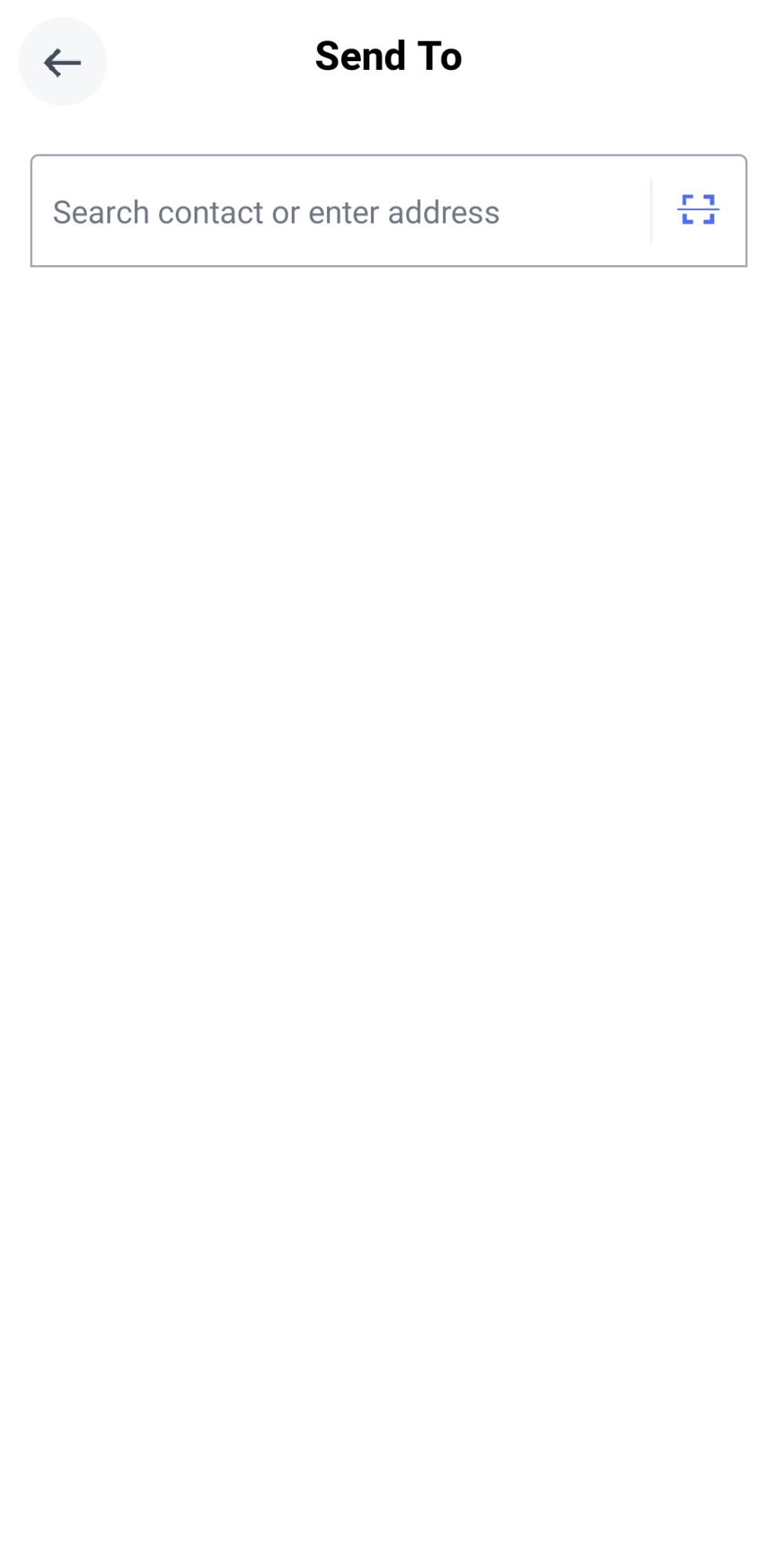The image displays a web or mobile interface graphic with a predominantly white background. At the top left corner, there's a faint gray circle containing a charcoal gray arrow pointing to the left. On the center of the screen, dark black capitalized text reads "Sent to the Essence", with the word "to" also capitalized. Directly below this text, there is a search bar outlined with a thin black rectangle. Inside the search bar, the prompt says "Search contact or enter address" with only the "S" in "Search" capitalized. Toward the right side of the screen, a light purple fine line is visible next to a blue-purple square with partially open sides, creating a box with breaks in the lines. The horizontal line through the middle of the square extends from east to west.